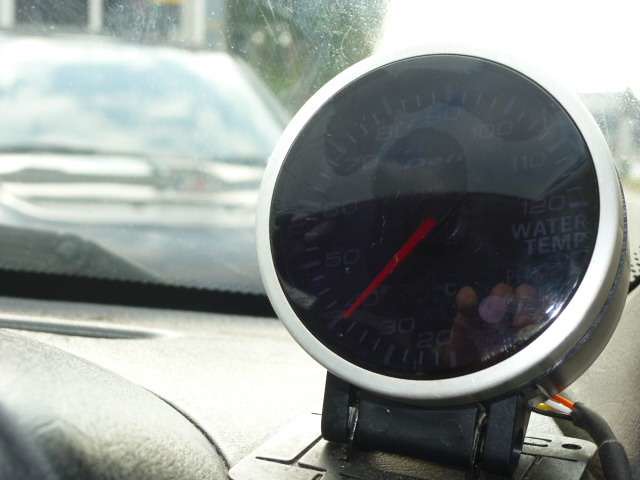The image captures the interior of a car from the driver's perspective. The dashboard is prominently displayed, featuring a water temperature gauge on the right side. The gauge is circular, slightly tilted backwards and upwards towards the camera, and has a silver rim with a glass cover. Inside, the gauge is black with white numbers running clockwise from 10 to 120, with "water temp" inscribed below the numerical scale. A red needle within the gauge points just below the 40 mark.

To the left of the gauge, a gray steering column is partially visible, arching up and over from right to left, with a slit in the dashboard above it, likely an air vent. The dashboard itself ascends to about halfway up, then angles slightly downwards to the right.

A black brace supports the gauge from beneath, resting on a small flat steel piece. Various wires—white, orange, yellow, and black—extend from behind the gauge, trailing into a black cover that disappears out of the frame at the bottom.

Through the somewhat dirty windshield, the front grille and bumper of another vehicle can be seen, with the bumper being black. Additionally, a portion of the driver's side windshield wiper is visible on the left side of the frame.